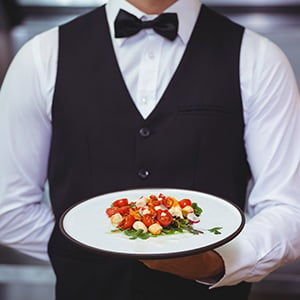The image features a close-up view of a fine-dining waiter, impeccably dressed in a white button-up long-sleeve shirt, a black vest with shiny buttons, a black bow tie, and a neatly pressed outfit. His right arm is elegantly folded behind his back, while his left arm is bent at the elbow, extending a white plate with a black rim towards the camera. The plate holds a beautifully arranged, colorful salad consisting of vibrant red tomatoes, white croutons or cheese, and assorted green leaves. The background is a vague blur of silver tones, emphasizing the sophisticated restaurant ambiance.